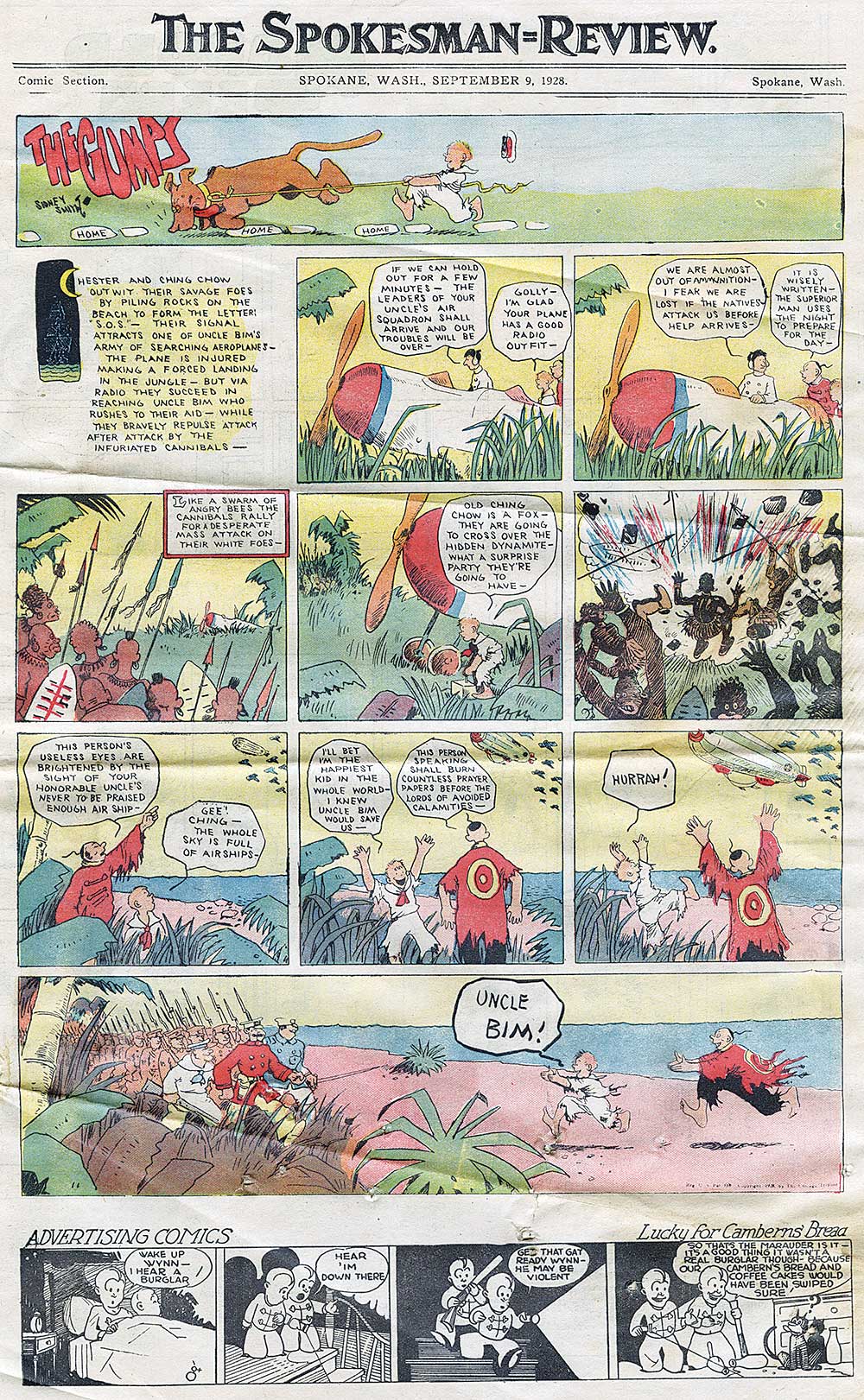This image features the comic section of a newspaper presented in a portrait-oriented rectangular layout against a white background. The topmost portion displays the name of the newspaper, "The Spokesman-Review," in black font, followed by smaller text identifying the section as the "Comic Section." Between these headers, a double line runs horizontally across the image. The dateline reads "SPOKANE, WASH., SEPTEMBER 9, 1928," with "SPOKANE, WASH." capitalized for emphasis.

The comic section consists of five rows of comics and a bottom row dedicated to advertising comics, rendered in black and white. The first comic at the top left corner is titled "The Gumps," highlighted in red. This panel features a cartoon drawing of a brown dog tugging its leash while a barefoot boy dressed in white clings onto it.

Proceeding downward, the next three rows each contain three panels arranged in a grid format, making a 3x3 layout. The first panel in the upper left has only text: "Chester and Ching Chow outwit their savage foes," followed by approximately eight lines of narrative text. The subsequent images portray a scene featuring an airplane in tall grass surrounded by people and numerous text boxes. 

The second row's panels depict interactions with "savages" characterized by dark-skinned individuals with minimal clothing, shields, and spears. The middle-right panel of this row contains an explosion scene. The final panel extends across the width of the section, illustrating British army men arriving from the left and encountering Chester and Ching Chow on a beach, with Chester exclaiming, "Uncle Bim."

The bottom row is labeled "Advertising Comics," featuring a promotional strip for Cambern's bread. It includes four smaller panels depicting children discussing their preference for the bread in a simplistic, advertisement-driven narrative.

Overall, the image is a detailed historical snapshot of a 1928 comic section from "The Spokesman-Review," showcasing both serialized storytelling and commercial advertisements in a traditional newspaper format.